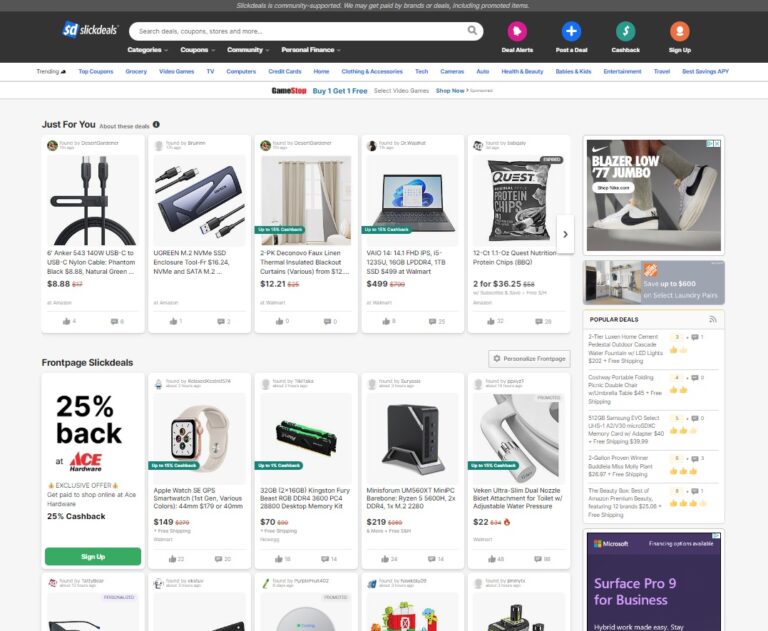The website displayed is "Slick Deals" (SD), a platform dedicated to finding and sharing the best deals. At the top, a prominent search bar allows users to search for deals, coupons, stores, and more. Just below, navigation options include Categories, Coupons, Community, and Personal Finance.

On the right-hand side, there are additional options such as Deal Alerts, List a Deal, Cash Back, and Sign Up. The main banner highlights trending deals in a rotating fashion, keeping users updated on the hottest offers.

The bulk of the webpage is divided into two main sections. The first section, labeled "Just For You," shows personalized deal recommendations. Each deal features an image, a brief description, and the current price. These suggested deals are tailored to the user's browsing history or preferences.

Below this is the "Front Page Slick Deals" section, showcasing popular deals with rectangular images. Each deal includes a picture, a brief description, the original price (which is crossed out), and the discounted price. For instance, one of the highlighted deals is an Apple Watch SE OPS smartwatch, featuring a clear image, a brief overview, the slashed original price, and the reduced sale price.

To the right, a sidebar contains advertisements, along with a list of popular deals indicated with thumbs-up icons and accompanying comments. This sidebar resembles a message thread, offering interactive elements for users to engage with the deals and community feedback.